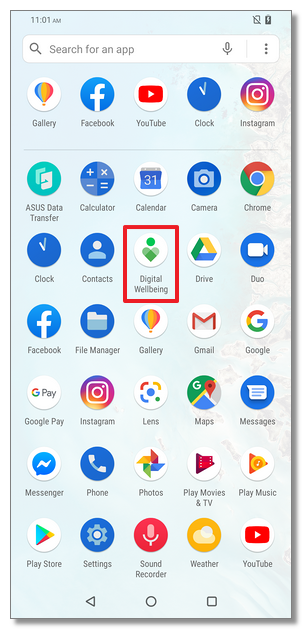The image depicts a smartphone screen with a light blue background and grey font. 

- In the top left corner, the time reads 11:01 AM.
- On the top right corner, there is a battery icon.

Below the status bar is a white search box with a grey magnifying glass icon to the left and a microphone icon on the right. There are also three dots, indicating more options.

The home screen icons are arranged in rows, starting with:

1. **Gallery**: Icon with a blue, orange, and red balloon.
2. **Facebook**: Icon showing the white "F" on a blue background.
3. **YouTube**: Icon featuring a red circle with a white play arrow.
4. **Clock**: Icon depicting a blue clock with white hands.
5. **Instagram**: Icon with a purple, yellow, and pink gradient background, a white outline, and a white circle in the middle.

Moving to the next row:

6. **ASUS Data Transfer**: Icon is a green circle with one white square and one green square.
7. **Calculator**: Icon displaying the plus, minus, multiplication, and equals symbols inside a circle.
8. **Calendar**: Icon showing 31 days in a blue box.
9. **Camera**: Icon of a grey camera with a white circle in the center.
10. **Chrome**: Icon displaying the Chrome logo with red, green, and yellow colors in a circle, with a blue dot in the center.

Further down:

11. **Clock**: Appears again with the same blue clock with white hands.
12. **Contacts**: Icon of a blue circle featuring a white head and shoulders.
13. **Digital Well-being**: Icon is a red square with a white circle and a green figure, possibly a heart.
14. **Drive**: Icon features a blue, green, and yellow triangle on a white background.
15. **Duo**: Icon is a blue circle with a white camera.

Next icons include:

16. **Facebook**: Reappears with the same white "F" on a blue background.
17. **File Manager**: Icon of a blue circle with what looks like a white and grey filing cabinet.
18. **Gallery**: Appears again with the same blue, orange, and red balloon icon.
19. **Gmail**: Icon depicting a red "M" on a grey and white background.
20. **Google**: Icon of a "G" in blue, red, yellow, and green on a white background.

Additional app icons include:

21. **Google Pay**, **Instagram**, **Lens**, **Maps**, **Messages**, **Messenger**, **Phone**, **Photos**, **Play Movies & TV**, **Play Music**, **Play Store**, **Settings**, **Sound Recorder**, **Weather**, and **YouTube**.

At the bottom of the screen:

- A grey triangle pointing left,
- A grey circle in the center,
- A grey square on the right.

This detailed description reflects the arrangement and design of each icon on the smartphone screen, providing a comprehensive visualization.